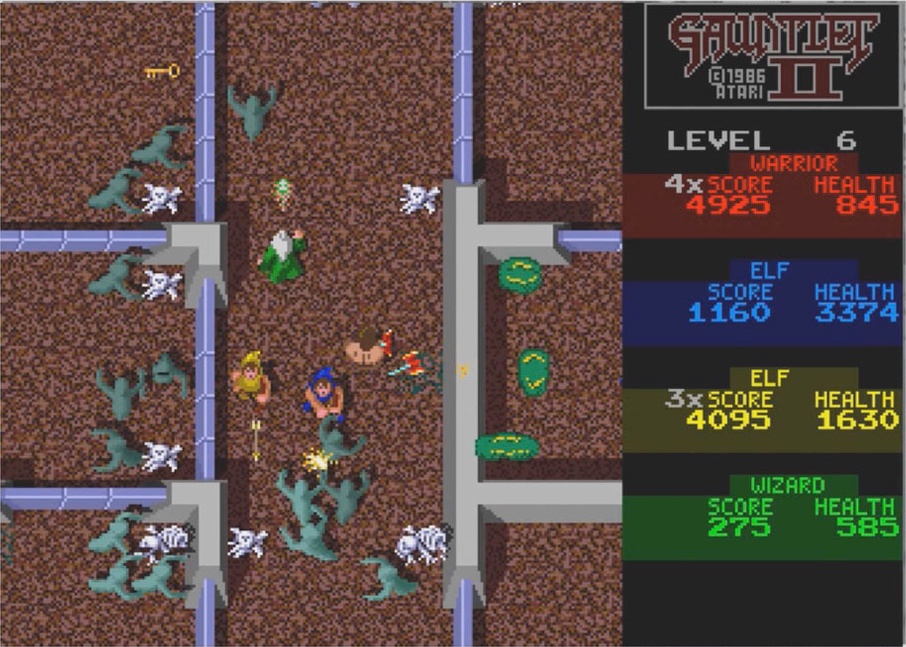This is a detailed screenshot of the classic computer game "Gauntlet II," developed by Atari in 1986. The upper left quadrant of the image features a black background with the title "Gauntlet II" prominently displayed; the word "Gauntlet" is rendered in a rust color, as is the Roman numeral "II." Beneath the title, in white text, is the current level indication: "Level 6," accompanied by the word "Warrior" in red. 

To the right is a statistics panel. It shows a "4x score" multiplier with the current score of 4,925 displayed in red. Below that, the player's health is shown as 845, also in red text. A separate black rectangle below these stats lists another score of 1,160 and a health value of 3,374, both written in blue.

The game also tracks multiple characters and their respective attributes. For instance, a yellow elf is confined to a rectangular box displaying a "3x score" multiplier (with "3x" in white and "score" in yellow) and a current score of 4,095. Next to this, the elf's health is listed as 1,630. Nearby, the stats for a wizard, shown in green text, list a score of 275 and health of 585.

The gameplay area depicts a grid-like maze resembling a tic-tac-toe board, with the center column occupied by a wizard. Characters including a yellow elf and a blue elf are engaged in combat against green monsters within the game's labyrinthine structure. Scattered around the maze are skull and bone graphics, notably at both the lower and upper center of the screen. Numerous monsters inhabit several of the rooms to the left, challenging the players as they navigate the game's intricate environment.